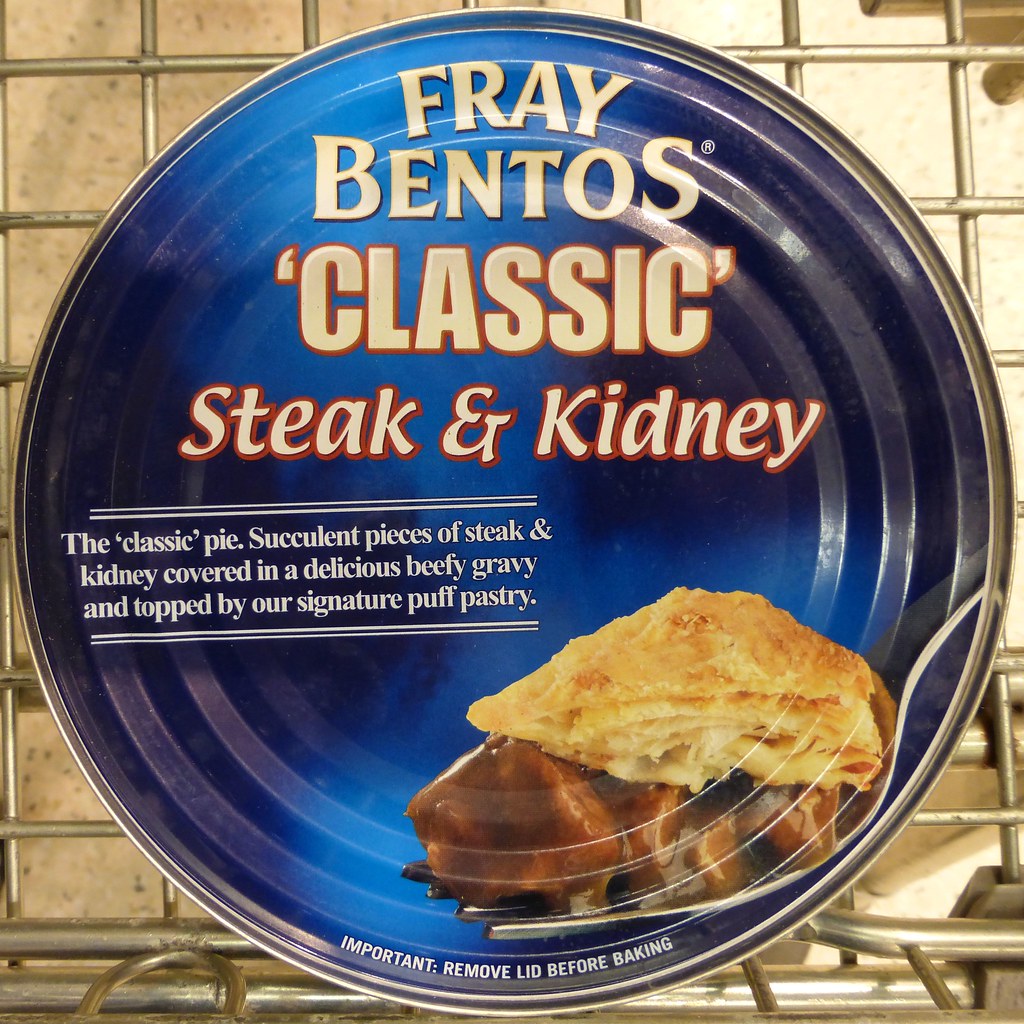The image features a blue can labeled "Fray Bentos Classic Steak and Kidney" resting on a metal cooling rack. The writing, "Fray Bentos Classic," is prominently displayed in beige with an orange border at the top of the can, followed by a description: "Succulent pieces of steak and kidney covered in delicious beefy gravy and topped with our signature puff pastry." A visual on the can shows a fork holding a piece of pie, with flaky puff pastry on top and beefy gravy dripping down. Notably, the can includes an important instruction, "Remove lid before baking." The metal cooling rack is positioned over what appears to be a marble countertop or flooring. The overall presentation emphasizes a ready-to-bake, savory pie encased in a silver-edged tin.